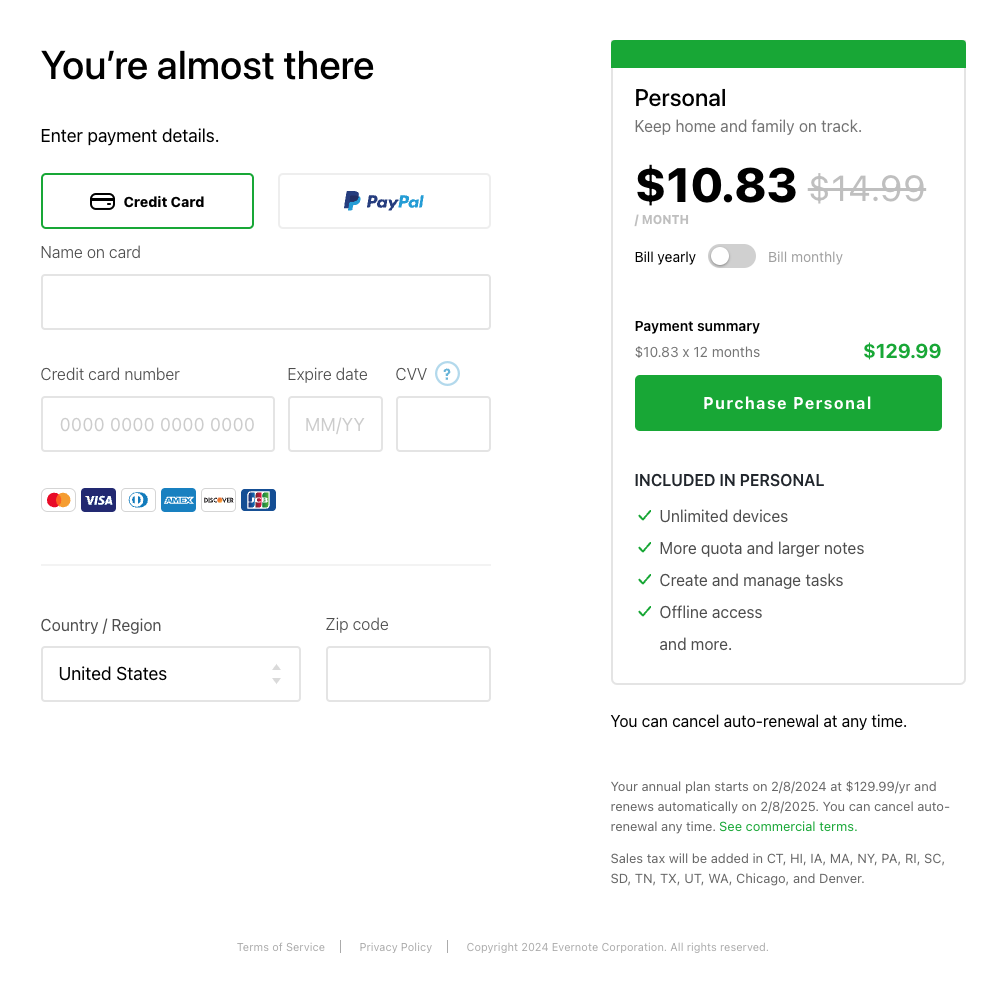In the upper left corner, the text "You're almost there" is prominently displayed. Below, the prompt reads "Enter payment details." Next to the outlined credit card in green, PayPal is also shown as a payment option. The form displays several fields, all currently blank: "Name on card," "Credit card number," "Expiration date," and a CVV field accompanied by a question mark within a circle. Beneath these fields, there is a list of accepted card logos including MasterCard, Visa, American Express, Discover, and two others whose icons are not identified.

A line labeled "Country or Region" displays "United States," and the "Zip Code" field remains empty.  

On the right side of the page, a green band marks the section dedicated to personal plan details. Below it, the heading reads "Personal: Keep home and family on track." The price is listed as $10.83 with an original price of $14.99 crossed out in gray. This is followed by the billing information showing the price billed yearly.  

Details of the payment break down to $10.83 per month, totaling $129.99 annually. At the bottom of this section, a green "Purchase Personal" button stands out.  

Included features of the personal plan are indicated by green check marks: unlimited devices, increased quota and larger notes, task creation and management, offline access, and more. It notes that you can cancel auto-renewal at any time. The plan's annual period will commence on 2/8/2024.